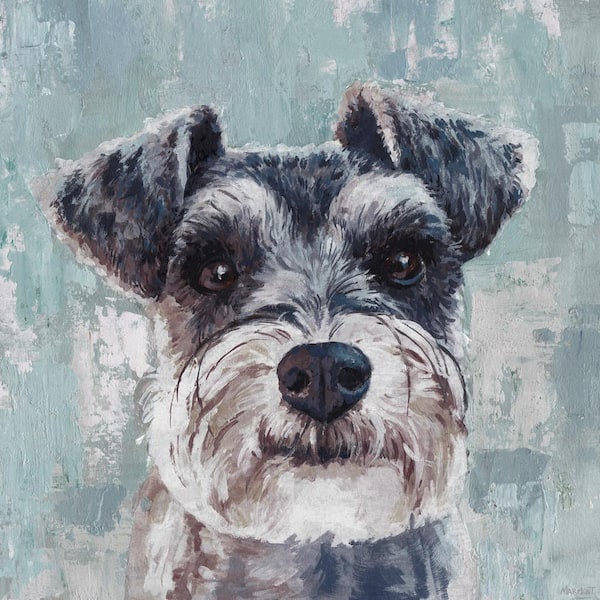The image is a meticulously detailed painting of a Schnauzer, depicted from the neck upwards. The square canvas showcases the Schnauzer's distinct features, including its gray fur with white accents around the mouth and nose forming a beard and mustache. It has noticeable black beady eyes and a black nose, with slightly gray eyebrows giving it a thoughtful expression. The Schnauzer's head is framed against a vibrant green background, which occasionally shows white spots and the textured ridges of layered paint, hinting at either acrylic or oil paint. The painting focuses solely on the dog's head, with its triangular, floppy ears adding to its charm. There is no text or artist signature visible on this artwork.